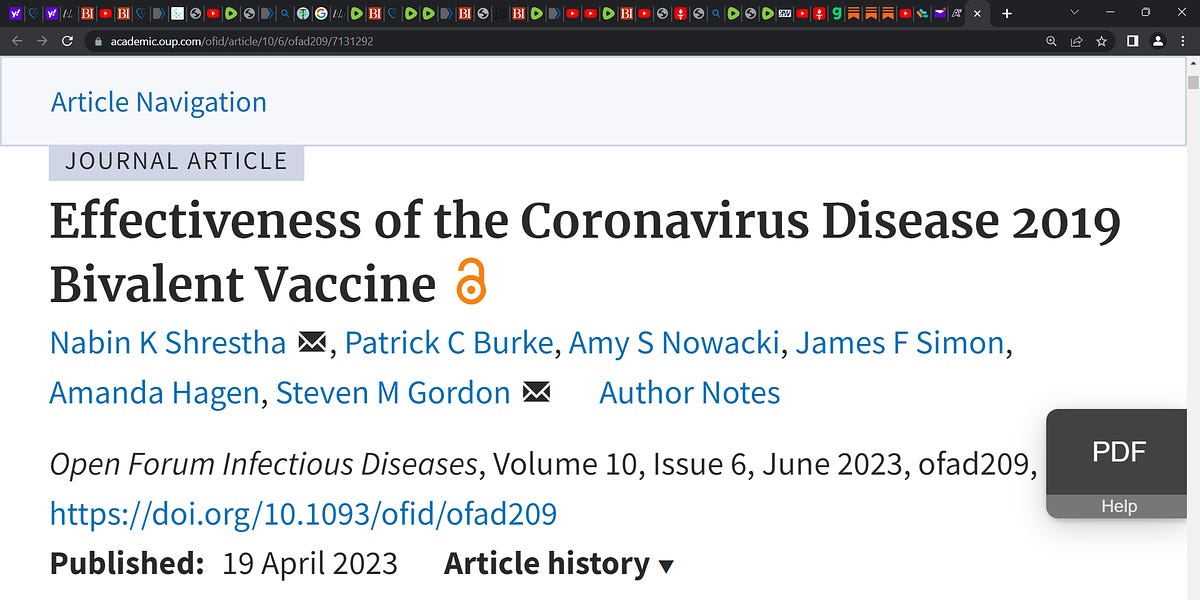This screenshot captures a detailed view of an academic journal article from a web browser. At the top of the screenshot, numerous tabs are open, suggesting extensive research or multitasking. Directly below, navigation tools including back and forward arrows, reload button, and an address bar are visible. The URL displayed is "academiccoop.com/OFID/article/10/6/OFAD209/7131292". Adjacent to the address bar, various icons are present, including a search icon, a possible download symbol, a star for bookmarking, a user profile icon, a rectangle icon, and a vertical ellipsis for additional menu options. A scroll bar is located on the far right.

Below the address bar, the blue text "Article Navigation" is prominently displayed. Beneath this, a gray banner reads "Journal Article" in black text. Following this, on a white background, the article title is printed in black: "Effectiveness of the Coronavirus Disease 2019 Bivalent Vaccine". An orange-gold lock icon, appearing unlocked, sits to the right of the title.

The authors are listed next, each separated by commas: Navin K. Shrestha (with a male icon after), Patrick C. Burke, Amy S. Nowacki, James F. Simon, Amanda Hagen, and Stephen M. Gordon (another male icon follows his name). To the right of these names, "Author Notes" appears in blue.

Further details of the publication are provided: "Open Forum Infectious Diseases, Volume 10, Issue 6, June 2023, OFAD 209". On the right, a dark gray rectangle with lighter shading at the top contains the label "PDF", and a small "Help" section below. Next, a DOI link is noted: "https://doi.org/10.1093/OFID/OFAD209". Under this, the publication date is specified as "Published: 19 April 2023". To the right, "Article History" is in bold, accompanied by a downward-pointing black triangle.